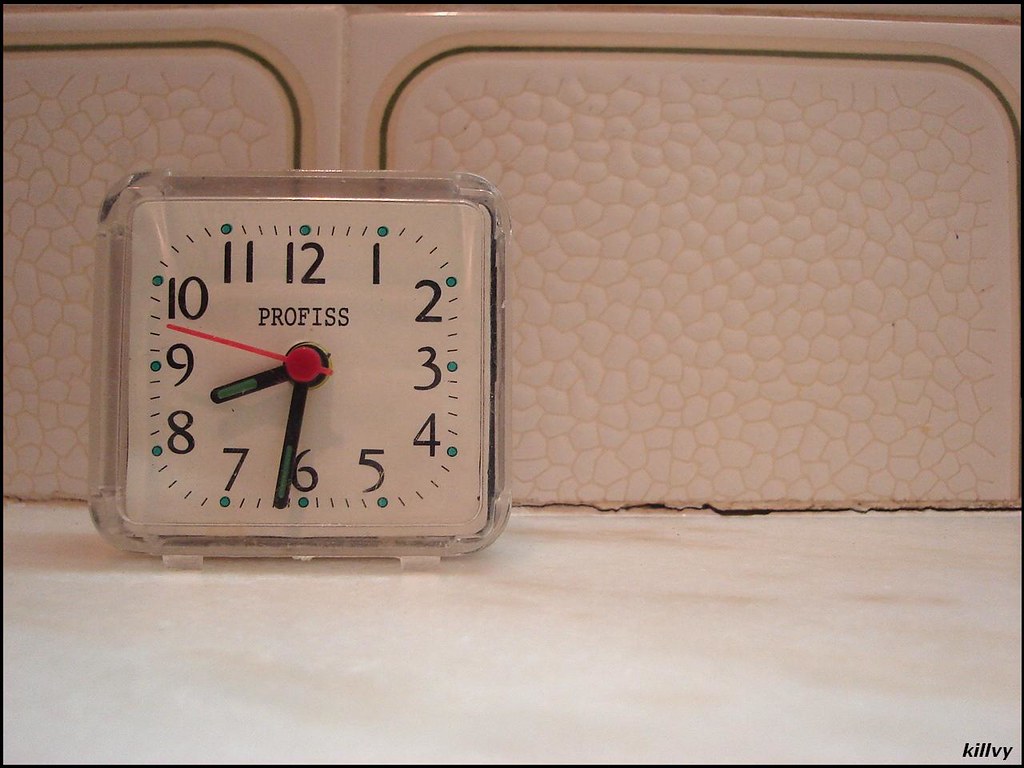The photograph captures a small countertop or desktop clock with a clear, likely acrylic or glass, casing and a square shape with rounded corners. The clock features a white face with black Arabic numerals, surrounded by teal (or blue) dots at each hour mark. Between the hour markers are small dashed lines signaling two-minute increments. The clock hands include a red second hand, as well as black minute and hour hands with blue stripes, possibly glow-in-the-dark. Above the clock hands and below the number 12, the maker’s name "PROFIS" is printed. The clock sits on a white surface. The backdrop is a ceramic-tiled wall with a white-orange peel texture, accented with thin green rounded square borders and standard white edges, though the grout is visibly imperfect, revealing jagged edges. The bottom right of the photograph is signed "KILLVY."